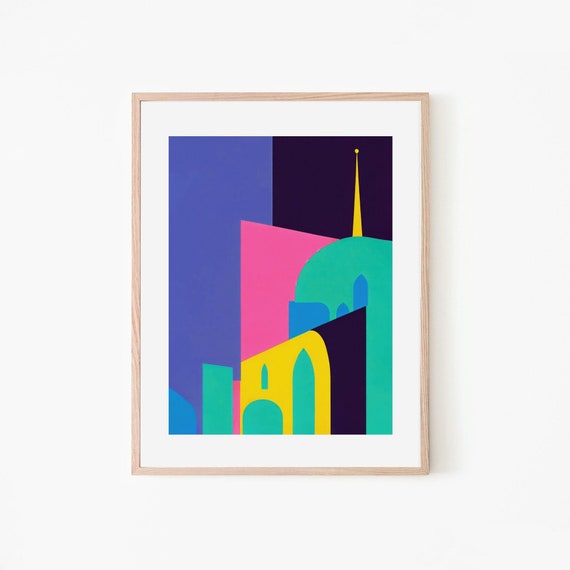This image is a photograph of a modern art painting, framed in a thin, light brown wooden border. Inside this frame is a white mat surrounding a vibrant depiction of abstract cityscape. The painting features large, colorful blocks and shapes, including a giant blue rectangle on the left and a pink rhombus in the center. At the bottom left, there are teal and blue squares, while the right side features a semi-circular green shape with a golden pointed steeple. The foreground includes yellow, black, and green skyscrapers, with a yellow antenna extending from a large green block at the top. The background is divided into shades of light and dark purple. The overall artwork is rendered in simplistic, block colors with no intricate details, highlighting its crude yet visually striking modern aesthetic.